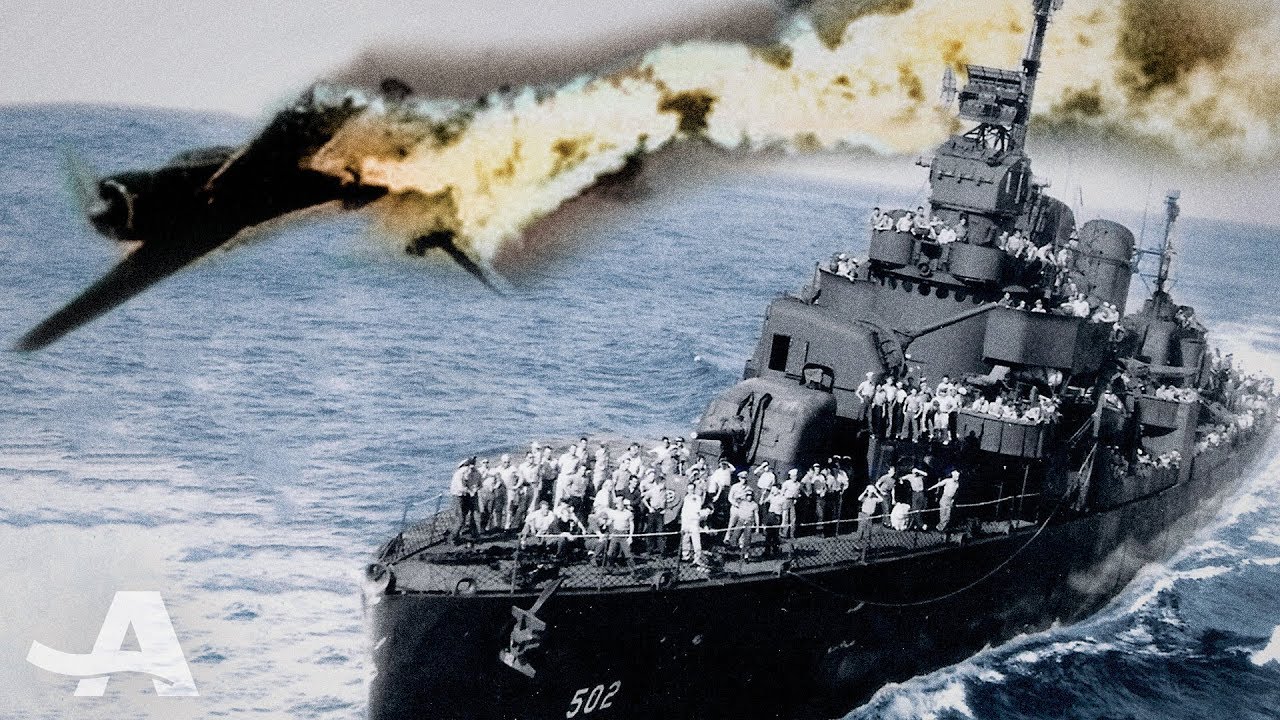The image depicts an imposing, large grey battleship situated on the right side of the frame. The ship, numbered 502 at the bow, has its anchor lifted and is filled with a large number of sailors, primarily men donning white navy uniforms, scattered across various deck levels as if posing for a photograph. The ship and its crew are rendered in black and white, emphasizing its vintage appearance. The waters surrounding the ship are a stark contrast in vivid blue, with subtle white waves created by the ship's presence. Dominating the backdrop is a photoshopped fighter jet or biplane, positioned at the upper left. The aircraft appears to have been hit, evidenced by an explosion on its tail, trailing yellow flames and orange smoke, and seems to be plummeting towards the ocean. The scene is an intriguing blend of old and new, accented by the letter "A" in the bottom left corner.